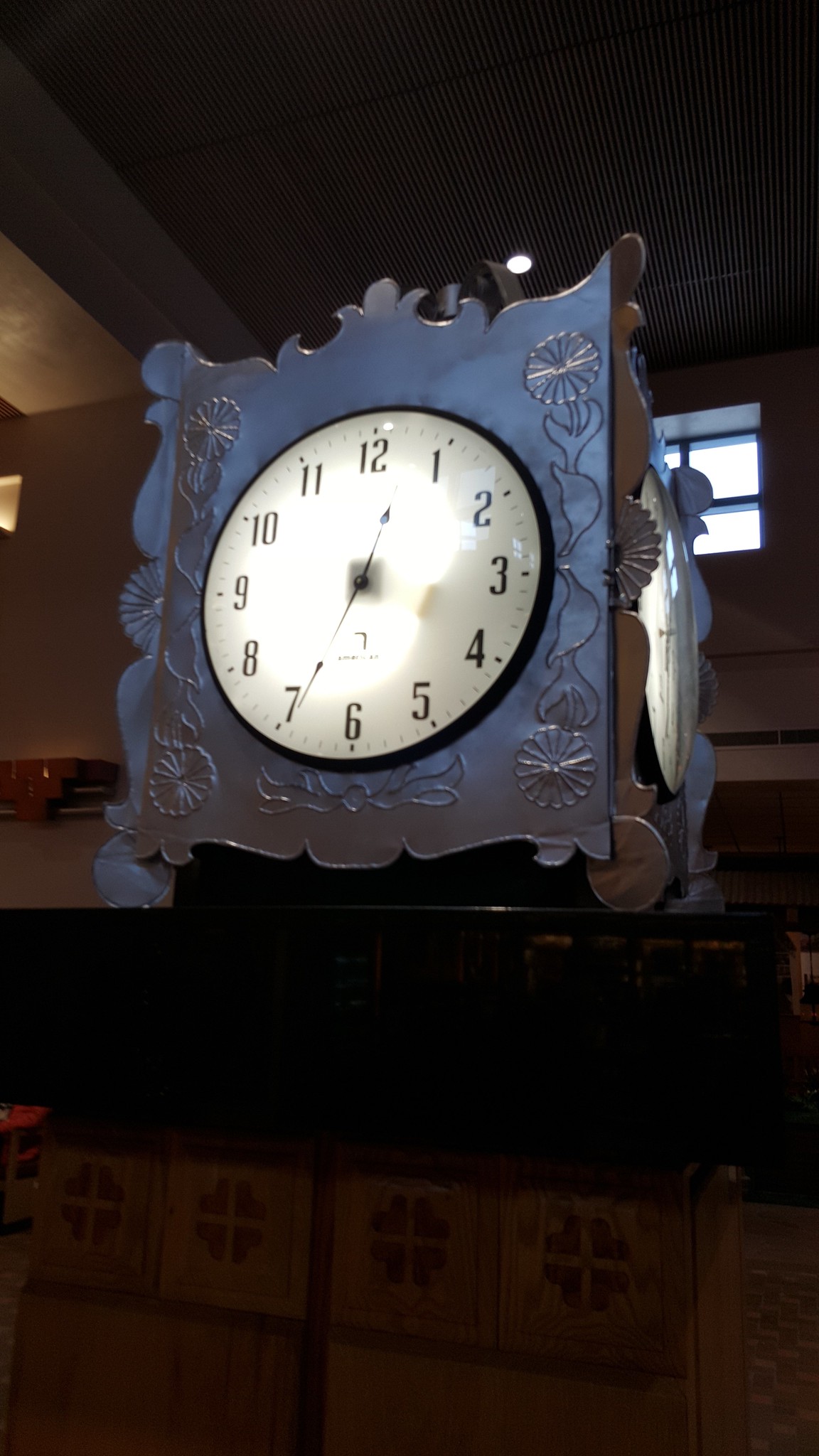The image depicts an antique clock with an ornate design, housed in a dark brown, metal box-like case. The round clock face is central and features black numerals on a glowing white background, displaying the time as approximately 12:35. On either side of the clock face, intricate flower and leaf motifs enhance its classic aesthetic. The clock, which evokes the size and shape of a protective shield, is resting on a table or shelf against a plank-style wall. The setting is indoors, with the top portion of a tan-colored wall and a small rectangular window visible in the background, along with a light fixture on the ceiling, suggesting the scene is part of a home or office interior.